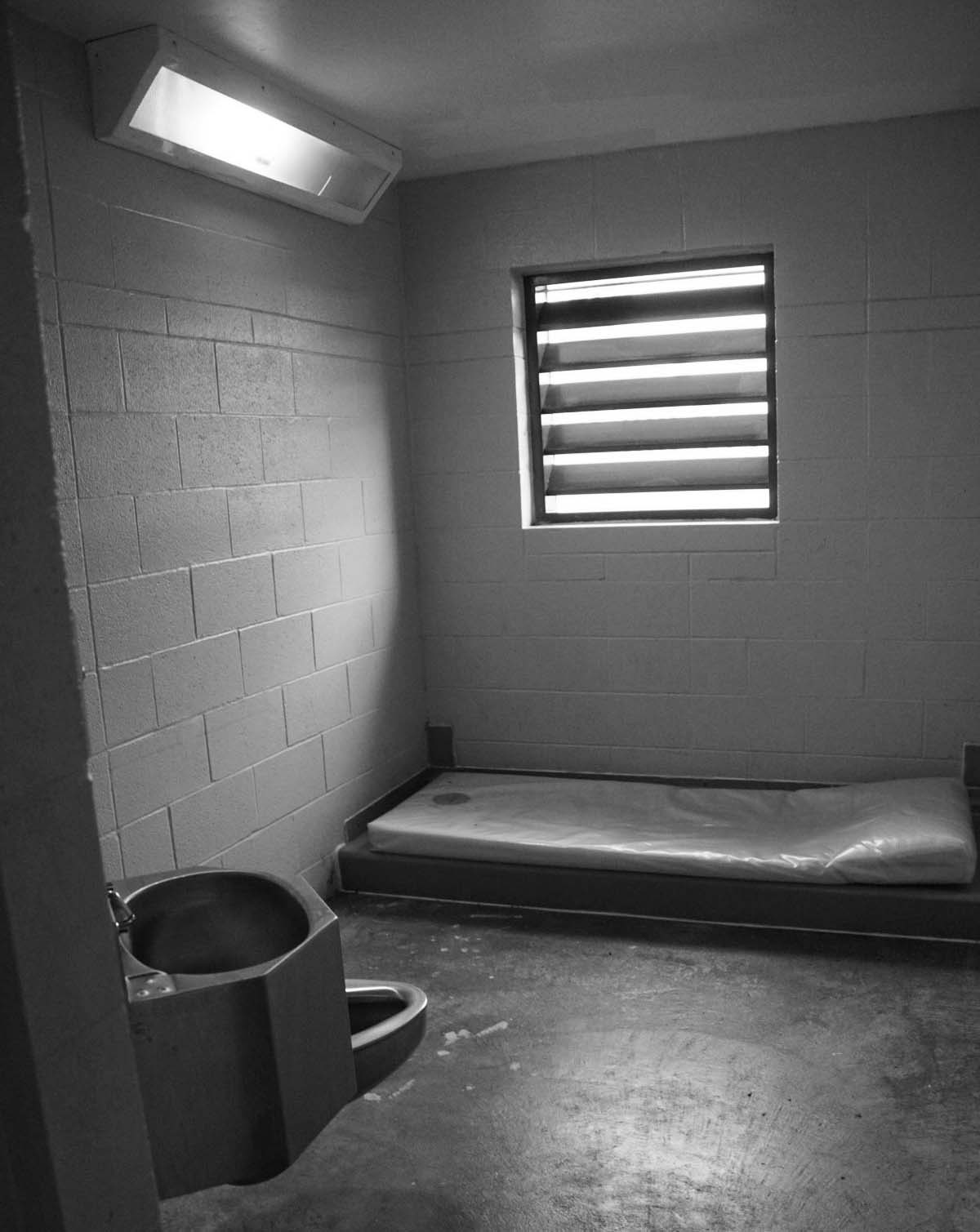The black and white image depicts a confined, desolate prison cell with sparse furnishings and a distinct sense of sterility. The cell is primarily constructed of light-colored cinder block walls: one on the left and one at the back. The back wall features a small, barred window with dark, horizontal slats that impede any clear view outside, allowing only minimal light to filter in. A fluorescent light fixture is mounted on the ceiling at the left side, casting a harsh glow over the space.

Situated against the back wall is a low-to-the-ground bed, consisting of a very thin, dark grey pad with a lighter grey pad on top, suggesting a built-in pillow area. This pad appears to be made of an easily cleanable material, likely plastic. The floor itself is plain, dark grey concrete, emphasizing the stark environment.

In the bottom left corner of the image, affixed to the wall, is a basic metal toilet without a lid, accompanied by a simple, compact sink. Both fixtures are made of silver metal, with the sink featuring a small faucet and a basic hole for water drainage. The toilet includes an arch-shaped protrusion further adding to the cold, utilitarian feel of the cell. Overall, the image captures the bare minimum amenities provided in this stark and unwelcoming incarceration space.